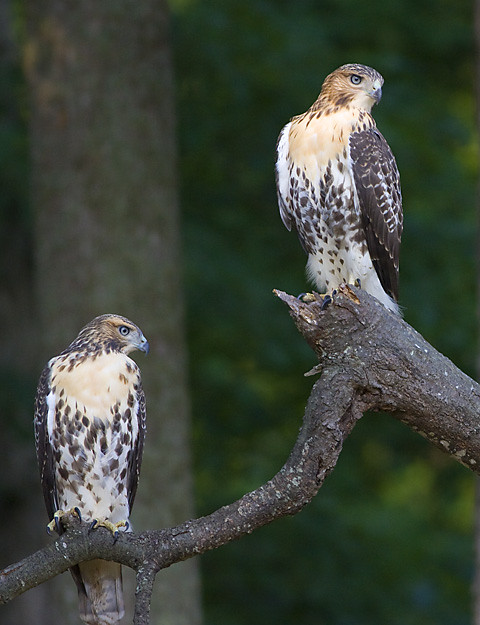This is a full-color outdoor photograph taken during the daytime. The background is a lush mix of green and yellowish hues, attributed to blurry trees and foliage, creating a soft, natural setting. On the left side of the image, one tree stands out clearly, showcasing its trunk without the dense cover of leaves.

In the foreground, a thick tree branch, appearing as though it has been cut or broken off, hosts two birds of prey. These birds, likely hawks, exhibit a striking plumage of white and brown. Their wings are predominantly brown, while their chests are white speckled with brown. The birds, perched at different heights on the branch, are both intently looking toward the right side of the picture. The branch itself is a typical brown color, with a noticeable broken part on the right side near where the rightmost bird is perched.